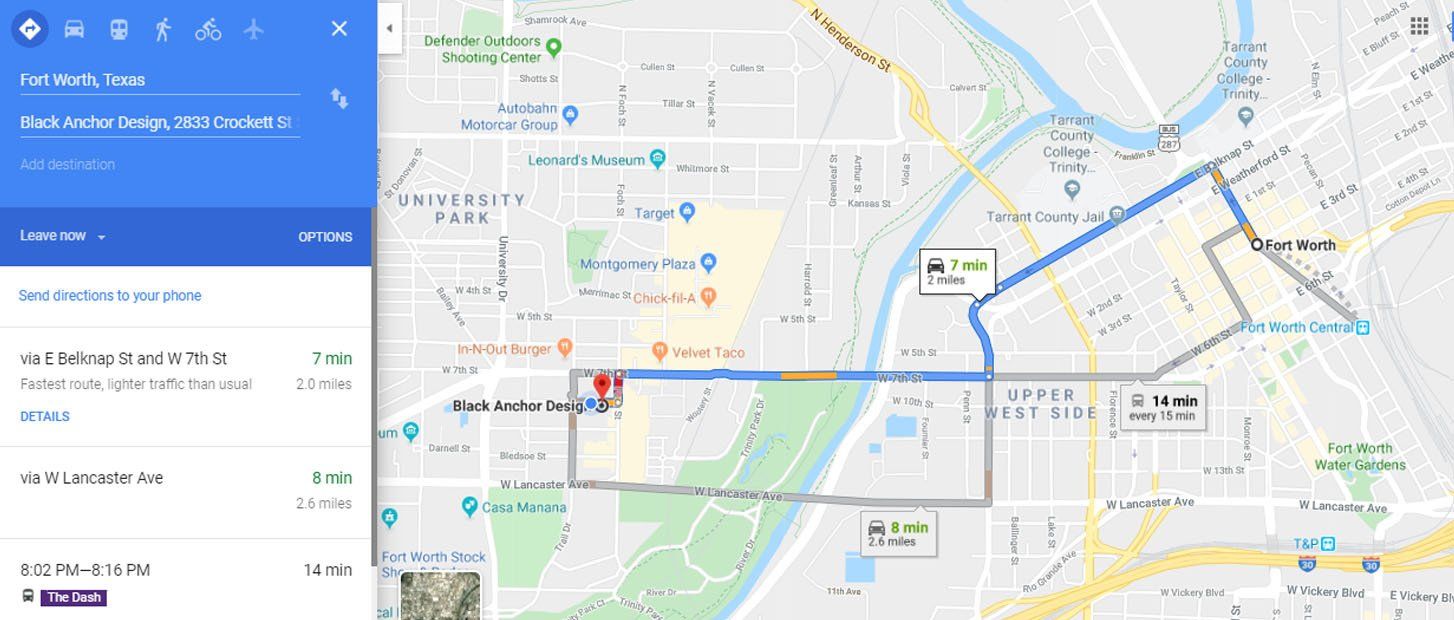The image displays a comprehensive view of a map interface. On the left side, an open page presents various navigational options. At the top half, set against a blue background, there are icons for different modes of travel including car, train, cycling, and plane. Below, a text box details the journey from Fort Worth, Texas to 833 Crockett Street, highlighting several intermediary stops such as Bank and Cartesan.

Further down, against a white backdrop, there are prompts to send directions to your phone, alongside an indication of the fastest route with lesser than usual traffic. Specific details outline the journey: it covers several miles along Lancaster Avenue, taking approximately 8 minutes to cover the 2.6-mile distance. The estimated travel time is from 8:02 PM to 8:16 PM, totaling 14 minutes.

On the right side, there's a detailed map showing the route from Fort Worth. The route, shaded in blue, begins near the Fort Worth Central and stretches to Black Anchor Design, which is near the In-N-Out Burger. The destination is marked with a red check location icon, clearly indicating the end of the journey.